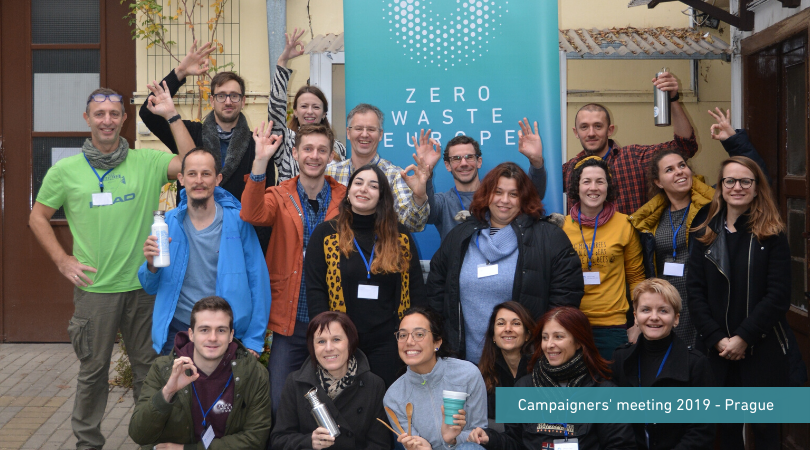In this lively group photo taken at the Campaigners Meeting 2019 in Prague, approximately 18-20 smiling individuals gather in front of a textured cream-colored wall adorned with plants and a prominent turquoise-to-blue gradient banner reading "Zero Waste Europe" with a white dotted logo. The bottom right corner of the image features the event's label in white text on a blue background. The participants, mostly dressed in long pants or jeans and long-sleeved shirts or jackets, exude a cheerful and positive energy, with many making the "OK" sign with their hands. Some wear glasses and lanyards with IDs, and a few hold various items like water bottles, a ceramic cup, and wooden spoons. The group is arranged in three rows, with six people in both the front and back row, and eight in the middle row. Notably, a person in the back row, dressed in a red and black plaid shirt, displays a stainless steel water bottle, while another individual in the middle row, wearing a blue jacket, holds a white water bottle. The brick pathway underfoot suggests they are outside, gathering for this memorable snapshot.